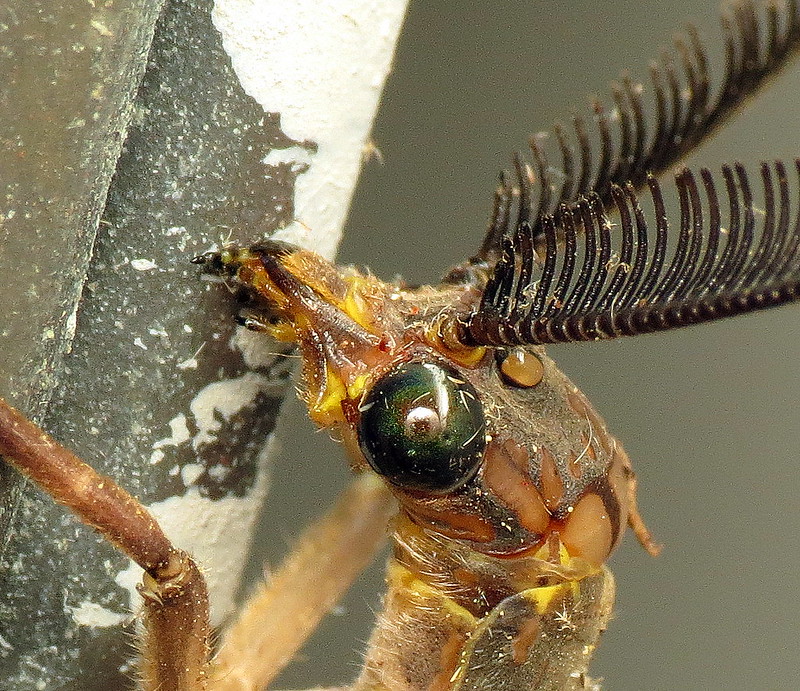This professionally staged, close-up outdoor photograph captures a fascinating insect in meticulous detail. Set against a blurred gray background, the image emphasizes the insect's unique features. The bug's body is predominantly brown and yellow, with long, comb-like black antennae resembling black plastic combs or feathered structures. Its head is tan to brown with a distinctive yellow and brown mouth that tapers to a needle-like tip, evoking the colors of a bumblebee. The insect is shown chewing on some material, possibly a mix of bark and other organic matter, which is brown and white. Prominently featured is the insect's huge, green eye with a central black or white color, adding vibrant contrast. A droplet of water is perched atop its head, while the back of its head displays an orange hue. Its segmented legs transition from brown to tan closer to the body and are covered in fine hairs. A metallic object with white patches and gray spots, possibly weathered and chipping, occupies the upper left part of the scene, adding a textured backdrop that highlights the intricate details of the bug.